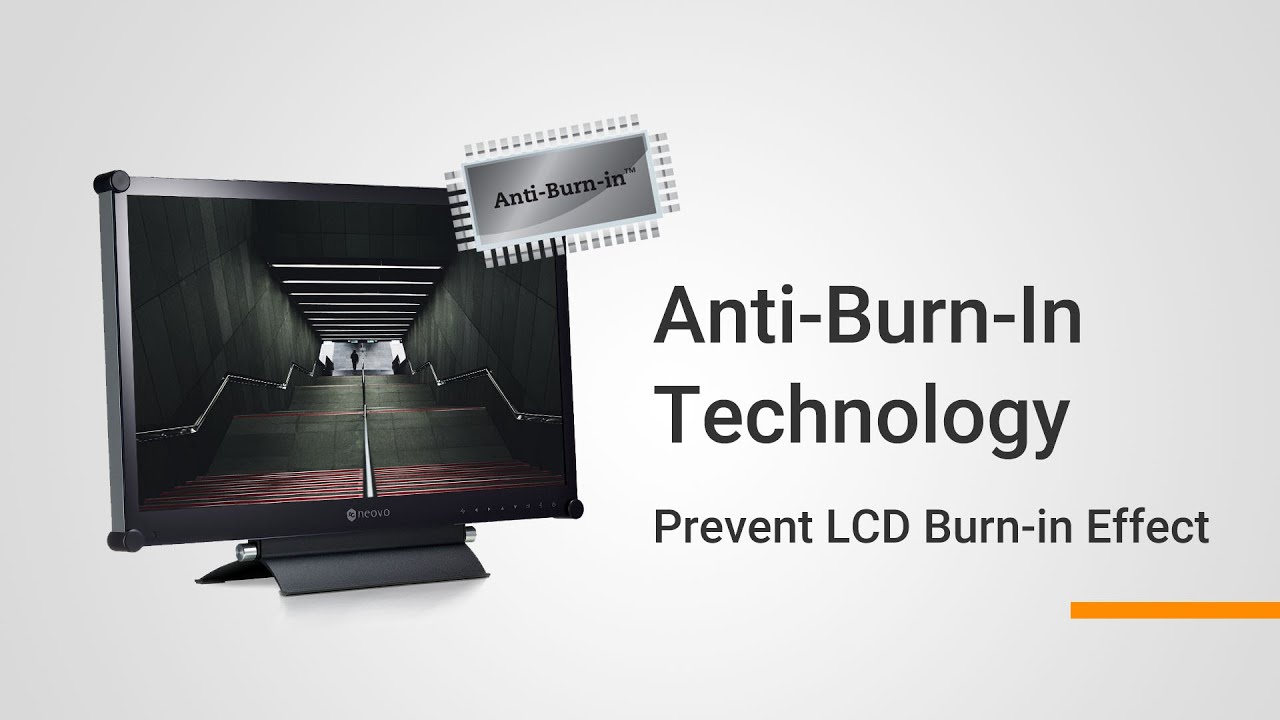The image showcases a detailed advertisement for anti-burn-in technology against a predominantly grayish background. On the left side of the image, a black monitor, approximately 17 or 18 inches in size, displays a high-definition picture of a person walking down a dark stairwell, creating a 3D-like depth effect. At the top right of the monitor, a silver and white sticker reads "anti-burn-in TM" and features a computer chip-like design. To the right of the monitor, in bold black letters, the text "anti-burn-in technology, prevent LCD burn-in effect" is prominently displayed. Below this text, a thin orange line runs horizontally across the image, emphasizing the advertisement for the anti-burn-in technology designed to prevent LCD screen burn-in effects.